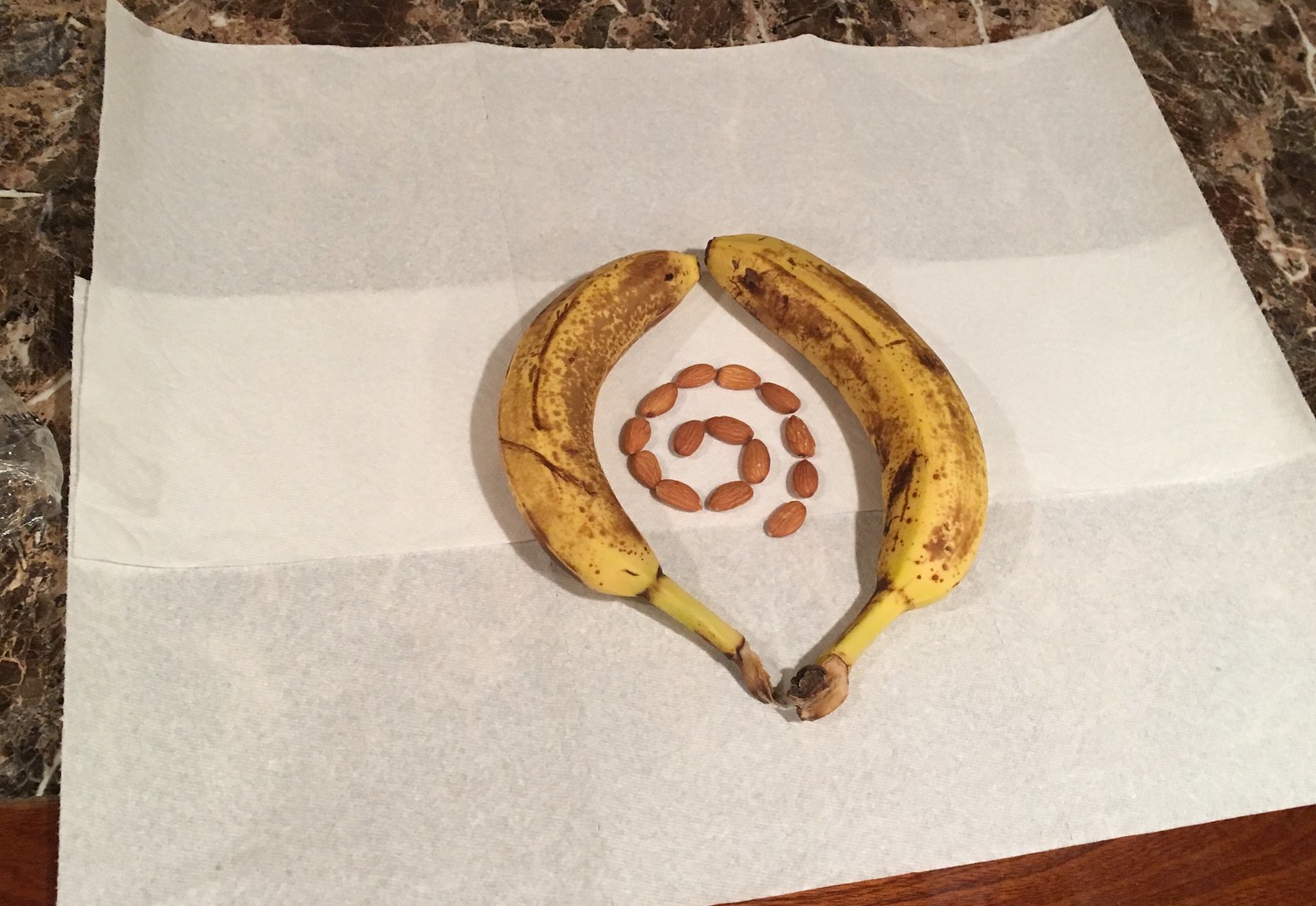The image captures an indoor scene featuring a granite countertop with a wooden base visible in the background. On the countertop, two white paper towels, slightly overlapping each other, create a brighter white area in the middle where they intersect. On top of these paper towels are two ripe, yellow bananas with numerous brown spots, and a slightly blackened area on the right-hand banana, indicating their ripeness. These bananas are positioned in a way that their stems touch and their curved ends meet, forming an oval shape, resembling an almond. At the center of this banana arrangement is a pattern of almonds, laid out in a distinctive spiral or swirl-like pattern that starts in the middle and extends outward, resembling the number six. The detailed arrangement highlights the intricate positioning of the bananas and almonds against the contrasting background of the white paper towels and the sleek granite surface.